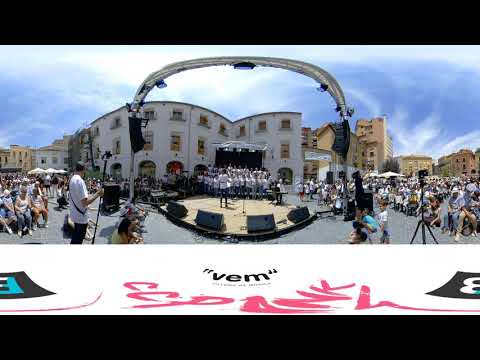This outdoor photograph captures a bustling concert scene in the middle of the day. A solid black border runs along the top and bottom of the image, framing the scene. Just above the lower black border is a white banner adorned with text in a foreign language, featuring discernible characters such as "V-E-M" in black, accompanied by some indistinct red writing.

At the center of the image is a tan-colored stage set against a backdrop of an outdoor plaza filled with a crowd of people, all dressed in summer attire like shorts and short-sleeved shirts, suggesting warm weather. On the stage, a group of performers stand in a line, uniformly dressed in white tops and blue bottoms. On the front edge of the stage, speakers are visible. An archway with lights frames the top of the stage, further illuminating the performers.

Flanking the stage on both sides, we see more spectators, adding to the lively atmosphere. The background showcases buildings—beige structures on the left and right, with a distinct white building in the center. Above these buildings stretches a blue sky dotted with clouds, completing this vibrant depiction of an outdoor concert venue.